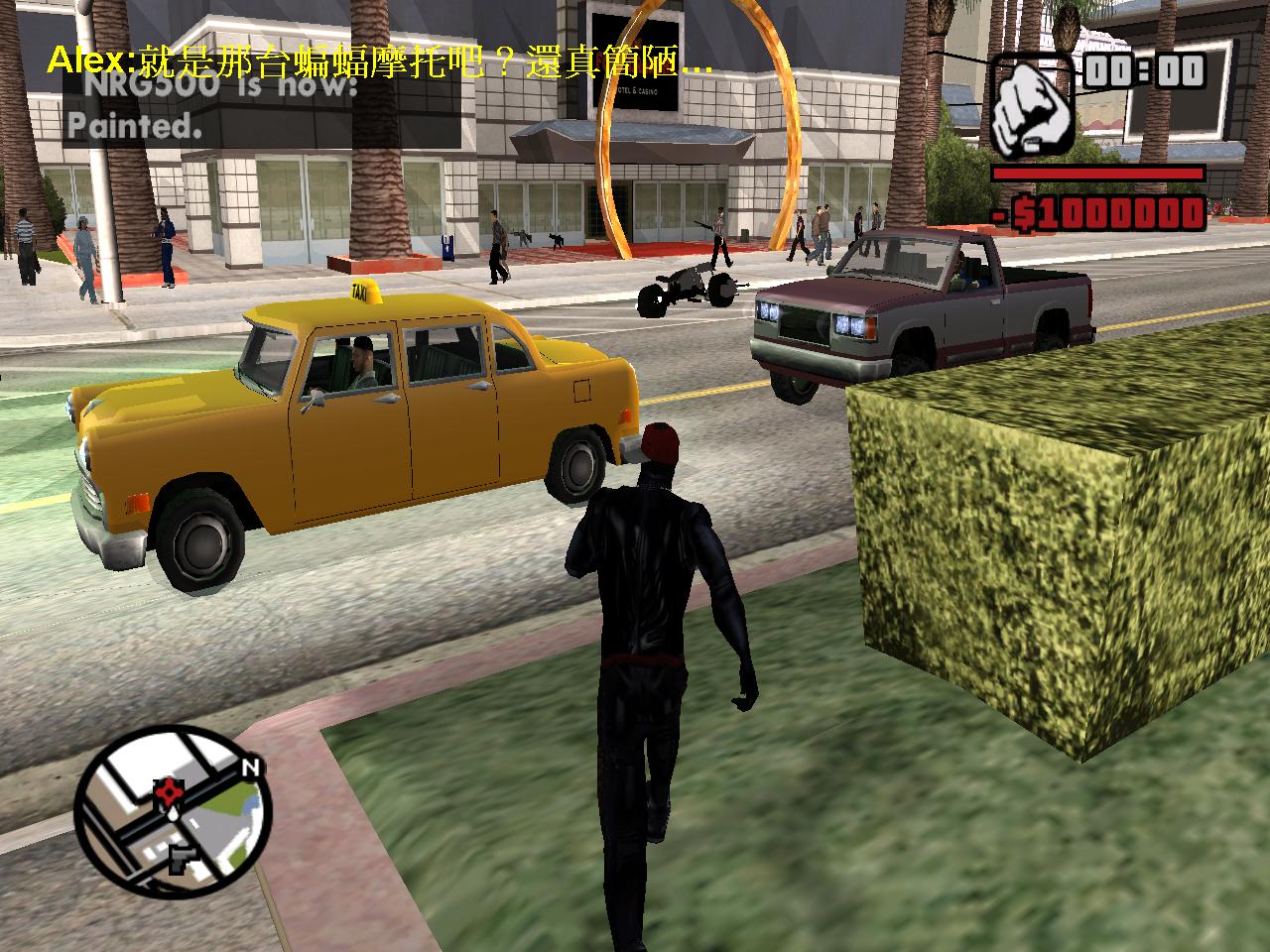In this rectangular nighttime scene from a video game, we observe a bustling city street that runs diagonally from the upper right to the lower left of the image. The street is crowded with people and vehicles. Dominating the lower left foreground, a yellow taxi cab with a driver wearing a black baseball cap is closest to the viewer. Directly behind the taxi is a gray and burgundy pickup truck, though its driver is not visible. 

On the opposite side of the street, slightly off-center, sits a black motorcycle parked in a no-parking zone. Adjacent to this motorcycle is a modern building with large glass windows, beyond which we can see a group of people, predominantly men, walking in both directions. 

In the upper left corner of the scene is what appears to be an office building, and printed in an Asian language is text we cannot decipher. Below this text, in gray print, it references "NRG 500 is now painted." The lower center of the image features the outline of a human figure walking away from the viewer.

At the very bottom left of the digital screen, there is a small circular minimap displaying the area’s street layout, aiding navigation in this elaborate virtual cityscape.